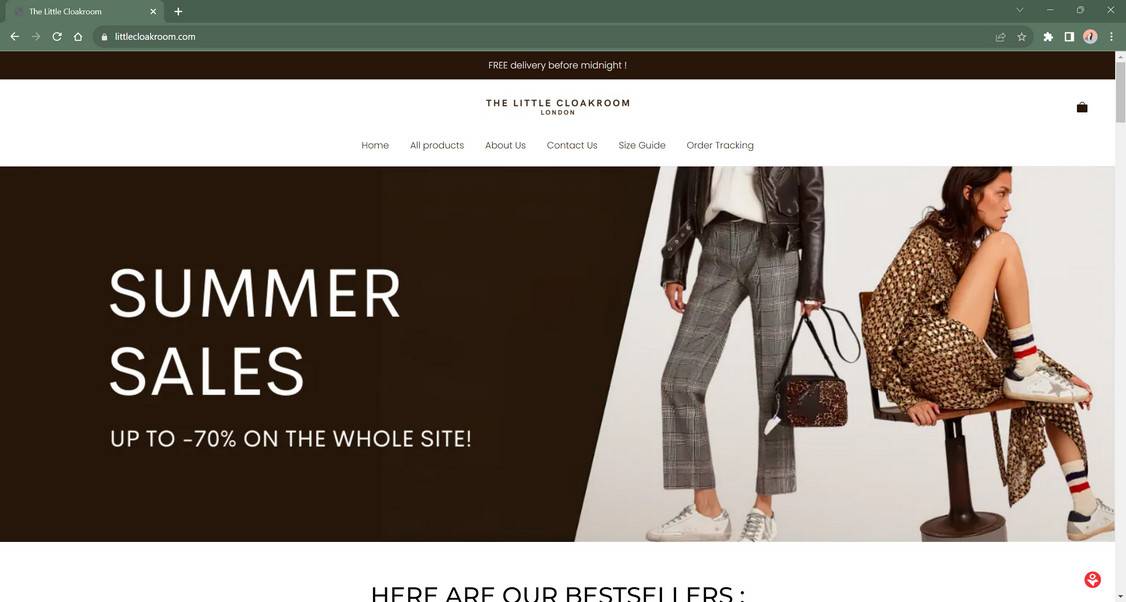Discover incredible deals with discounts up to 70% off site-wide at The Little Cloak Room! Featured here are our best sellers: A stylish individual dons gray plaid pants, a sleek leather jacket, a crisp white shirt, matching white shoes, and carries a chic brown purse. Beside them, a woman sits gracefully on a wooden chair with a black base, showcasing her unique style. She wears a distinctive brown dress with a scale-like, copper-toned texture. Her relaxed pose features one knee up on the chair, with her chin resting on her knee. Completing her outfit are white socks accented with blue and red stripes, paired with classic white tennis shoes.